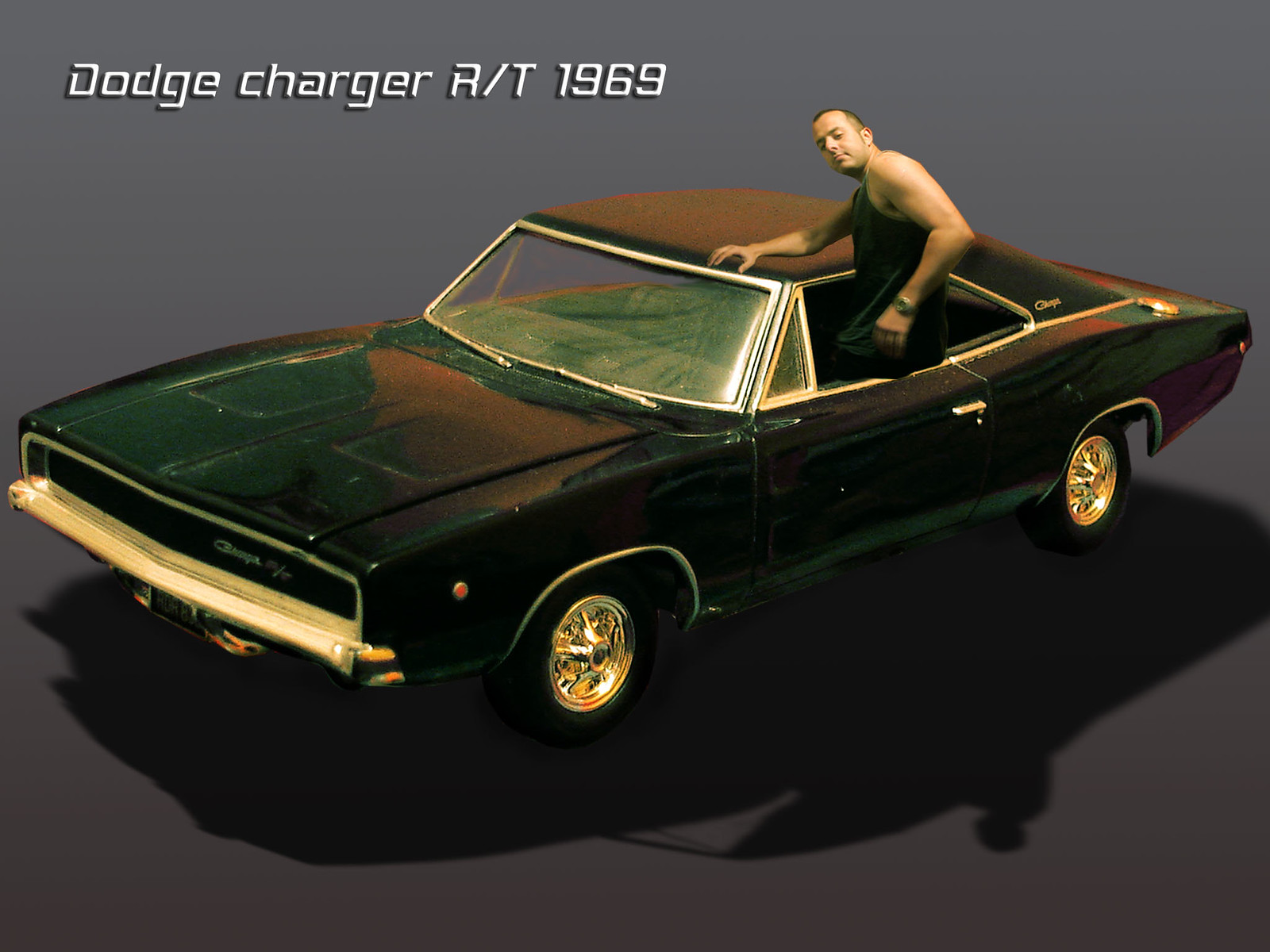The image is a digitally edited rectangular artwork featuring a black, 1969 Dodge Charger R/T with gold or silver details. The car, which has a black roof and a somewhat diagonal tilt with the front end pointing downward, is centered against a gray background. Beneath the car, a shadow adds depth to the composition. In the top left corner, the text "Dodge Charger R/T 1969" is displayed in italicized gray font. A Caucasian man with light skin, short buzzed black hair, and a dark tank top is seen seated in the driver's seat, hanging out of the window as his legs remain inside. He rests his right arm on the car's roof and sports a watch on his left wrist. The man appears to have been digitally inserted into the scene, contributing to the overall sense of Photoshop manipulation in the artwork.